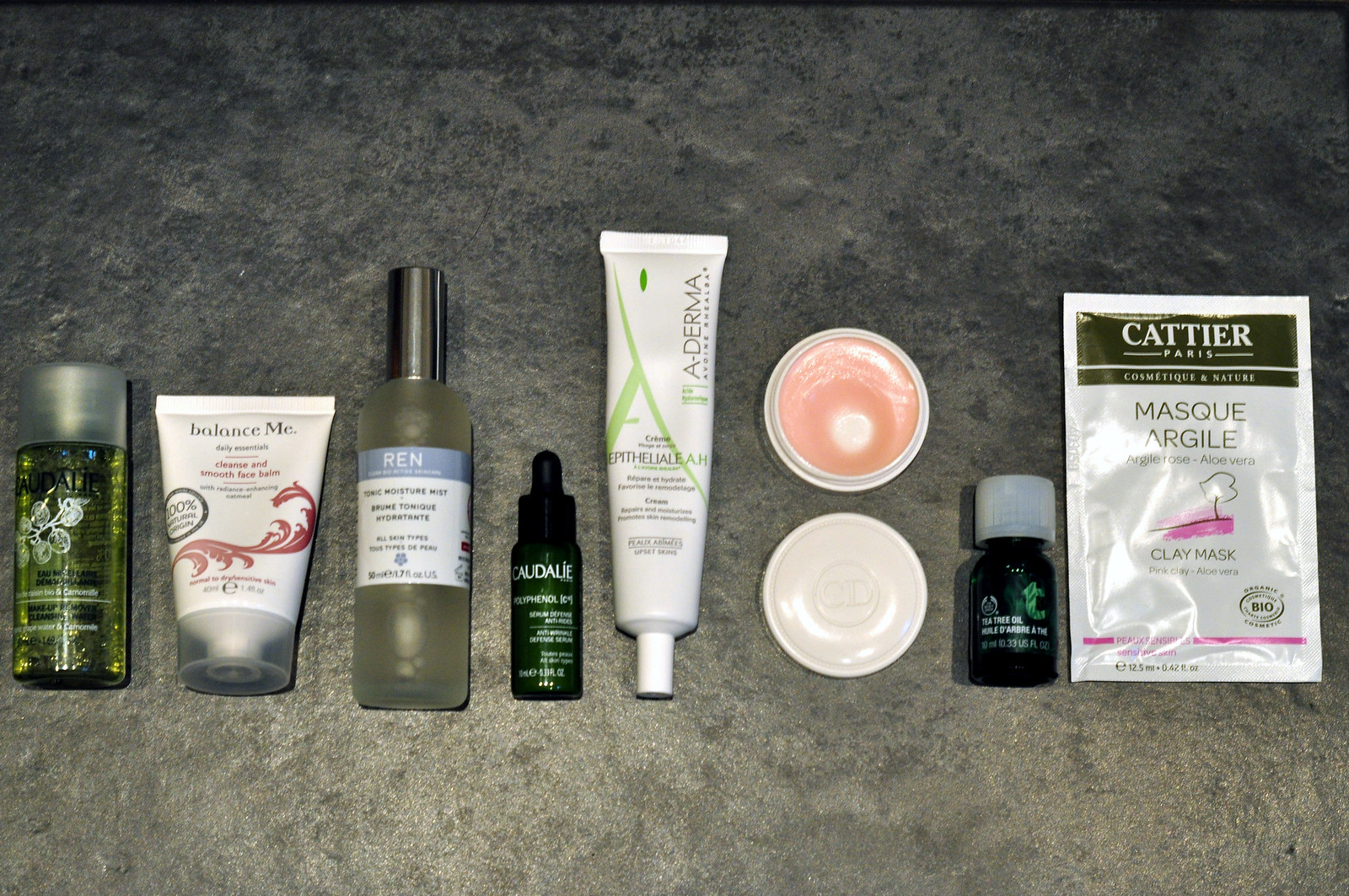In the image, a variety of self-care items are meticulously displayed. The first item is a light green bottle with a plastic cap, suggesting a soothing, perhaps organic product. The second item is a white container of cream labeled "Balance Me," complete with a clear plastic cap, indicating it might be for skincare balance and hydration. The third item is an elegant glass bottle with a shiny silver cap, prominently featuring the brand name "REN," hinting at a luxurious liquid skincare product. The fourth item is a bottle with a dropper, suggesting it may contain a serum or essential oil. The fifth item is a facial cream from the brand "A-Derma," with the words "epithelial something" visible on the packaging, resembling an upside-down white toothpaste tube. Additionally, an open jar of cream or wax is included, alongside a mysterious small black bottle. Lastly, a plastic package labeled "mask" is identified as a clay mask, integral for deep skincare routines.